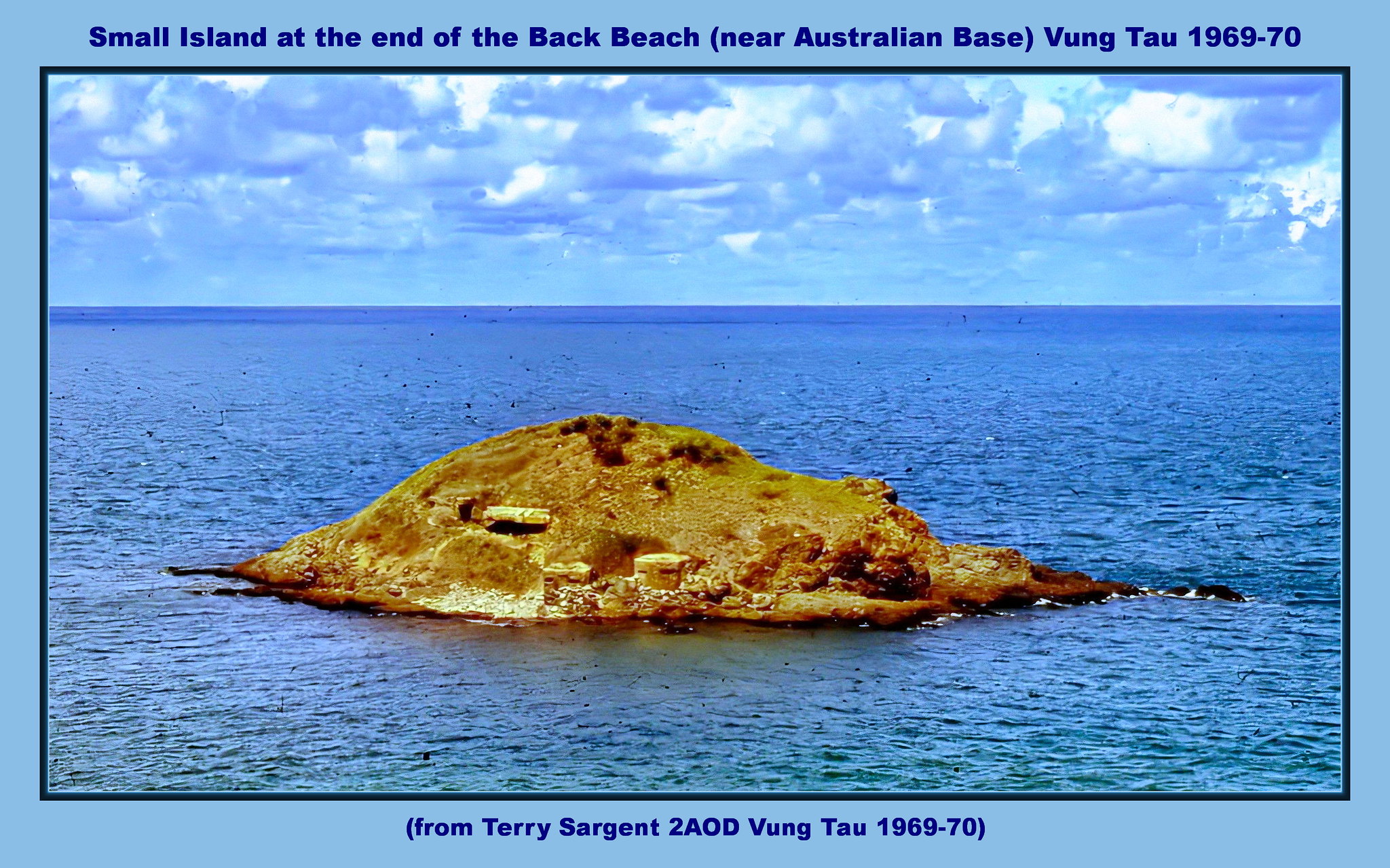This photograph, bordered by a light blue frame with a black outline, captures a daytime oceanic scene. At its center, a small, brown, hump-shaped island stands alone in the slightly choppy waters. The island lies under a blue sky accented with fair weather white clouds. The water is free of other objects, emphasizing the island's solitary presence. The text within the border reads, "Small island at the end of the back beach (near Australian base Vung Tau 1969 to 1970)." Below the image, it is credited, "From Terry Sargent to AOD Vung Tau 1969 to 70." The scene suggests an outdoor setting in Vietnam, likely near an Australian military base during the late 1960s to 1970. Colors such as light blue, dark blue, gray, white, brown, and tan dominate the tranquil yet historic snapshot.